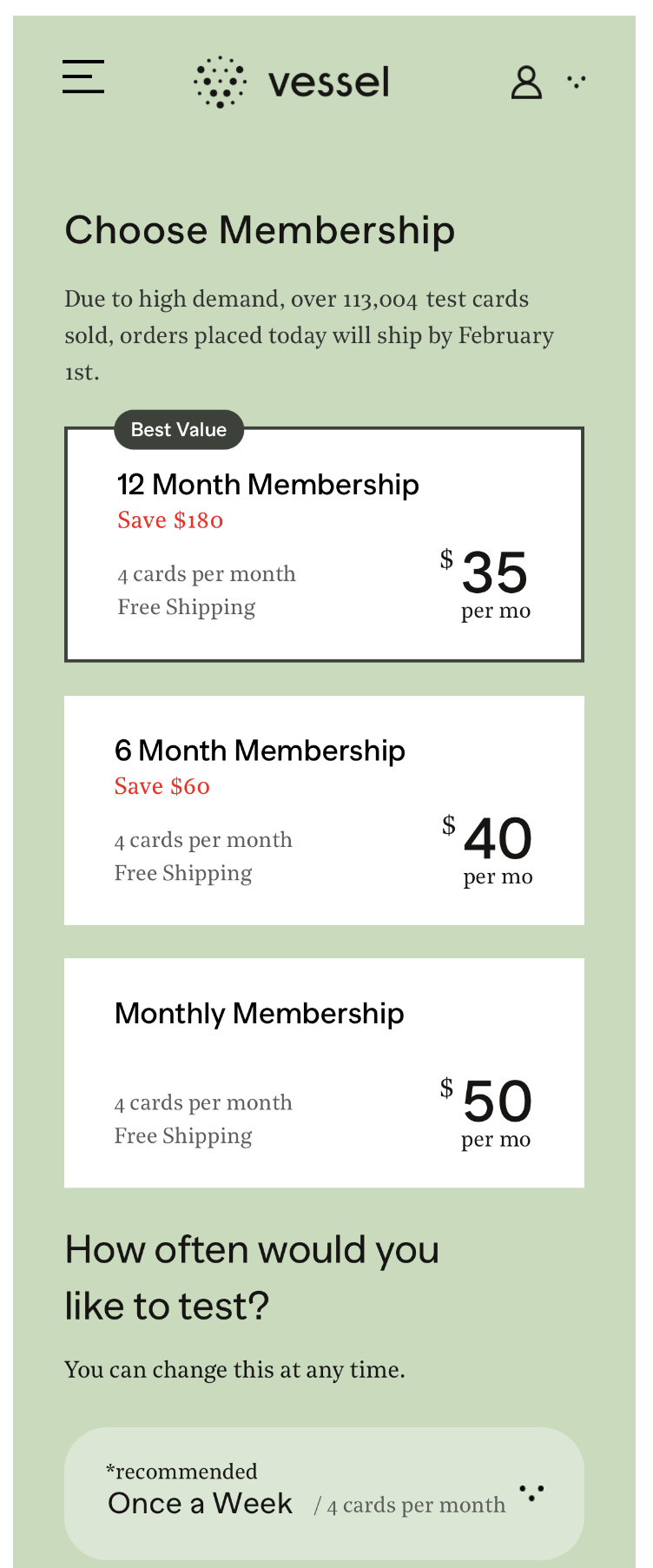The image displays a screenshot set against a white background, featuring a predominantly pale green interface. In the upper left corner, there is a vertically stacked three-line menu icon. Centrally positioned is bold black text reading "Vessel," accompanied by a circular logo composed of polka dots to its left.

Below "Vessel," bold black text reads "Choose Membership," followed by an announcement stating, "Due to high demand, over 113,004 test cards sold. Orders placed today will ship by February 1st."

A series of membership options are presented in white rectangular boxes. The first box is marked with a black button labeled "Best Value." This option is for a 12-month membership and emphasizes a savings of $180, with the "Save $180" text highlighted in red. Details include "four cards per month, free shipping, $35 per month."

The second option lists a six-month membership priced at $40 per month. 

The last option is for a Monthly Membership at $50 per month.

Below these options, against the green background, black text asks, "How often would you like to test? You can change this at any time."

The layout and design elements emphasize ease of navigation and clarity of choices, guiding the user through their membership options effectively.